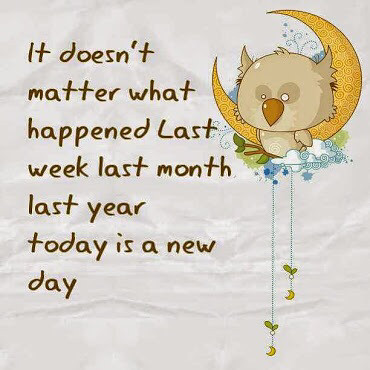In this image, we see a square poster or plaque with an inspirational message on a rough, mottled light gray background. The text, written in a yellow or goldish color and appearing hand-drawn but rendered by a computer, reads: "It doesn't matter what happened last week, last month, last year. Today is a new day." There are no punctuations in the statement. On the right side, there's an illustration of a light brown owl with an uneven appearance—one eye larger than the other—perched on a branch. The owl has a dark gold or yellow beak and stands against a yellow crescent moon. Below the owl, two stylized clouds are visible, and from the clouds hangs a pair of blue strings adorned with leaves and small crescent moons.